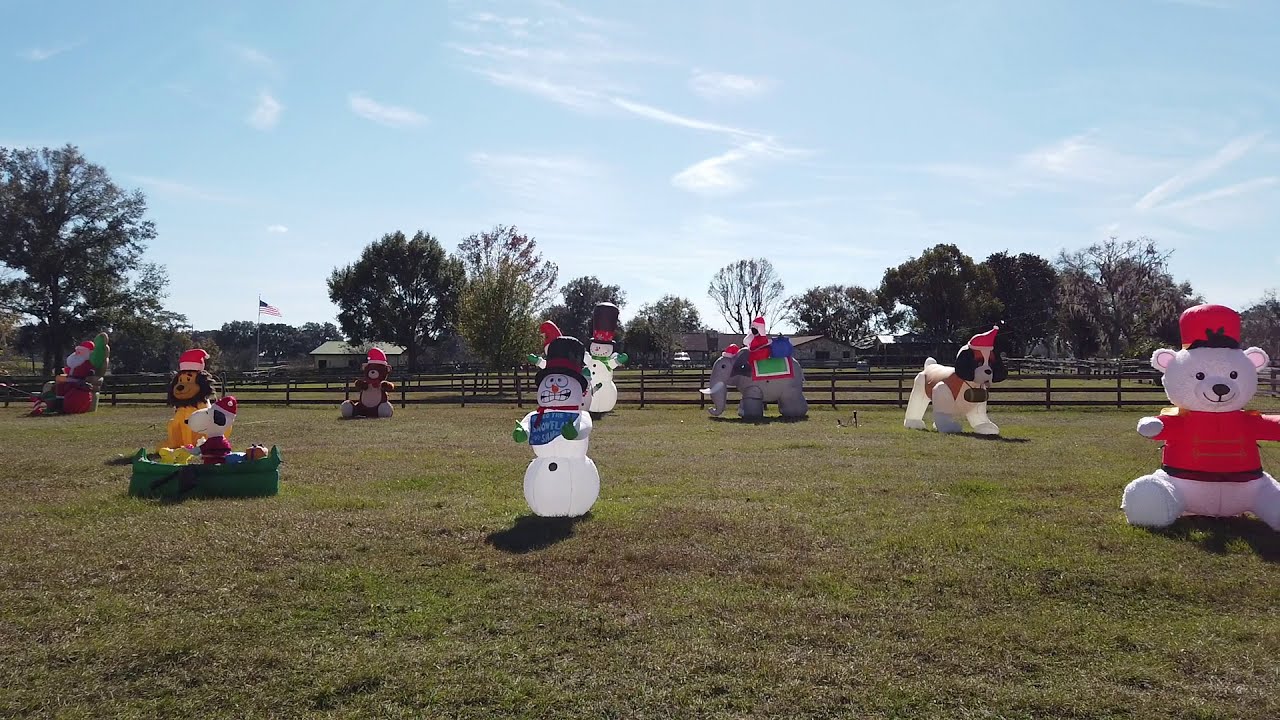In this vibrant outdoor scene taken on a bright, sunny day, a wide field is adorned with a collection of festive inflatable characters. The background features a clear blue sky with wisps of cirrus clouds and a tree-lined horizon, separated by a picturesque split-rail fence. At the forefront, central to the image, stands a prominent inflatable snowman donning a black top hat and a blue scarf. 

To the right of the snowman, there is a jolly white inflatable teddy bear in a red sweater and a matching tall red cap, smiling warmly. Further right, an inflatable dog with floppy brown ears, possibly a Boston Terrier, wears a Santa hat and clutches a present in its mouth. Near this dog, a Santa Claus appears to be riding atop an inflatable elephant, adding to the whimsical holiday display.

On the left side, adjacent to the snowman, is an inflatable lion sporting a Santa hat. Behind the lion, smaller in size, is an elf or gnome, standing tall. In the distance, another smaller inflatable bear can be seen, though its details are less distinct. Additionally, a Snoopy inflatable, seemingly in a green canoe, adds to the playful variety.

At the far left, a Santa Claus figure is positioned with a Christmas tree behind him. The entire scene exudes holiday spirit against the serene backdrop of trees and open grass, with occasional hints of nearby structures and an American flag peek through, bringing a festive touch to this tranquil rural landscape.